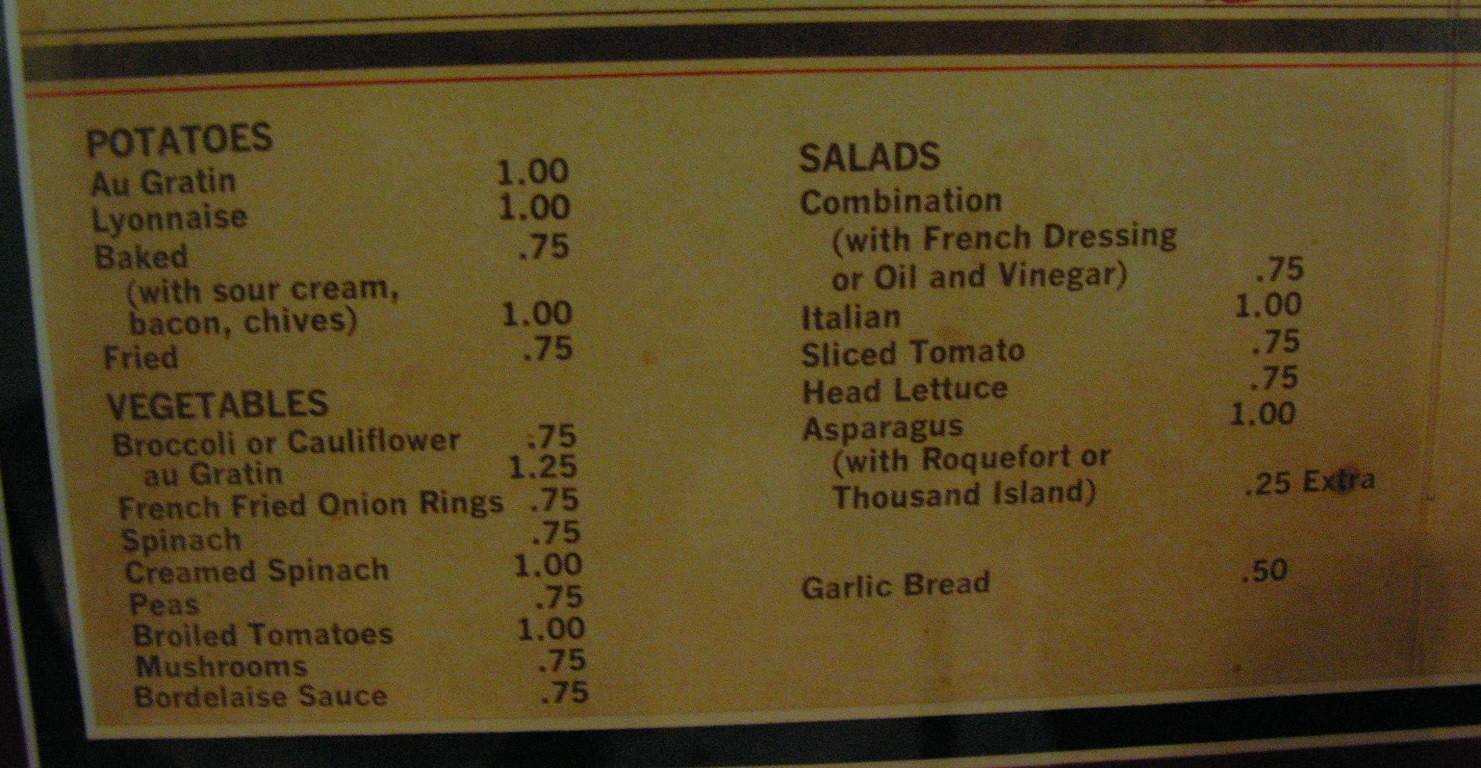The image presents an up-close view of a rectangular menu, showcased in a slightly off-center zoom. The background is a harmonious blend of beige, antique yellow, and cream shades, lending it a textured and dimensional feel. The menu is bordered by a modest black strip at the bottom left and right edges, though the exact location remains indiscernible, suggesting a setting within a restaurant.

Prominent black text stands out against the intricate beige backdrop. At the top, there's a thin red strip followed by a thicker black band, framing the details of the menu. The headings are in bold black, with the first section titled "POTATOES" in all caps. Listed underneath in a smaller, non-caps font are the varieties: "au gratin," "Lyonnaise," "baked with sour cream, bacon, and chives," and "fried," each accompanied by their respective prices on the right.

Following this, the heading "VEGETABLES" is displayed, with various types and their prices listed below. The final section, titled "SALADS," maintains a similar format with a heading in black and the salad options along with their prices listed beneath. The menu layout seems meticulously designed to be both detailed and organized, enabling easy reading and selection.